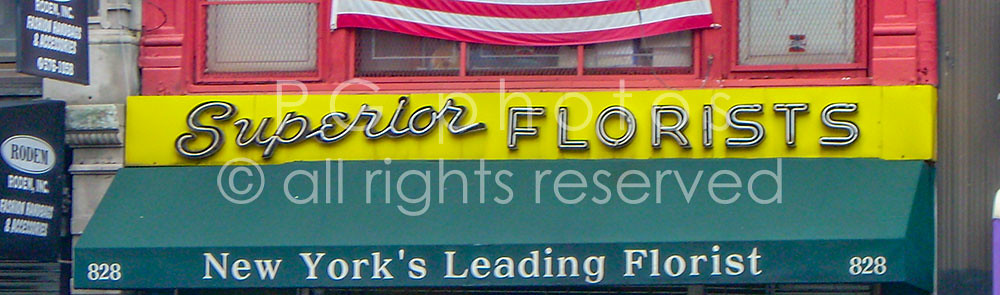The storefront of Superior Florists is featured prominently with its vibrant yellow facade. The name "Superior" is gracefully displayed in cursive script, while "Florists" is assertively written in block capital letters. A green awning extends across the front, bearing the address "828" in bold white numbers along with the tagline "New York's Leading Florist." The number "828" is also repeated on the right and left sides of the awning for added visibility. Above this, a red window facade can be seen, flanked by the bottom edge of an American flag, adding a touch of patriotic flair. The main building boasts a grey stone facade, providing a stark yet complementary background to the colorful storefront. The image has a watermark reading "PG Photos copyright, all rights reserved," ensuring proper credit to the photographer.